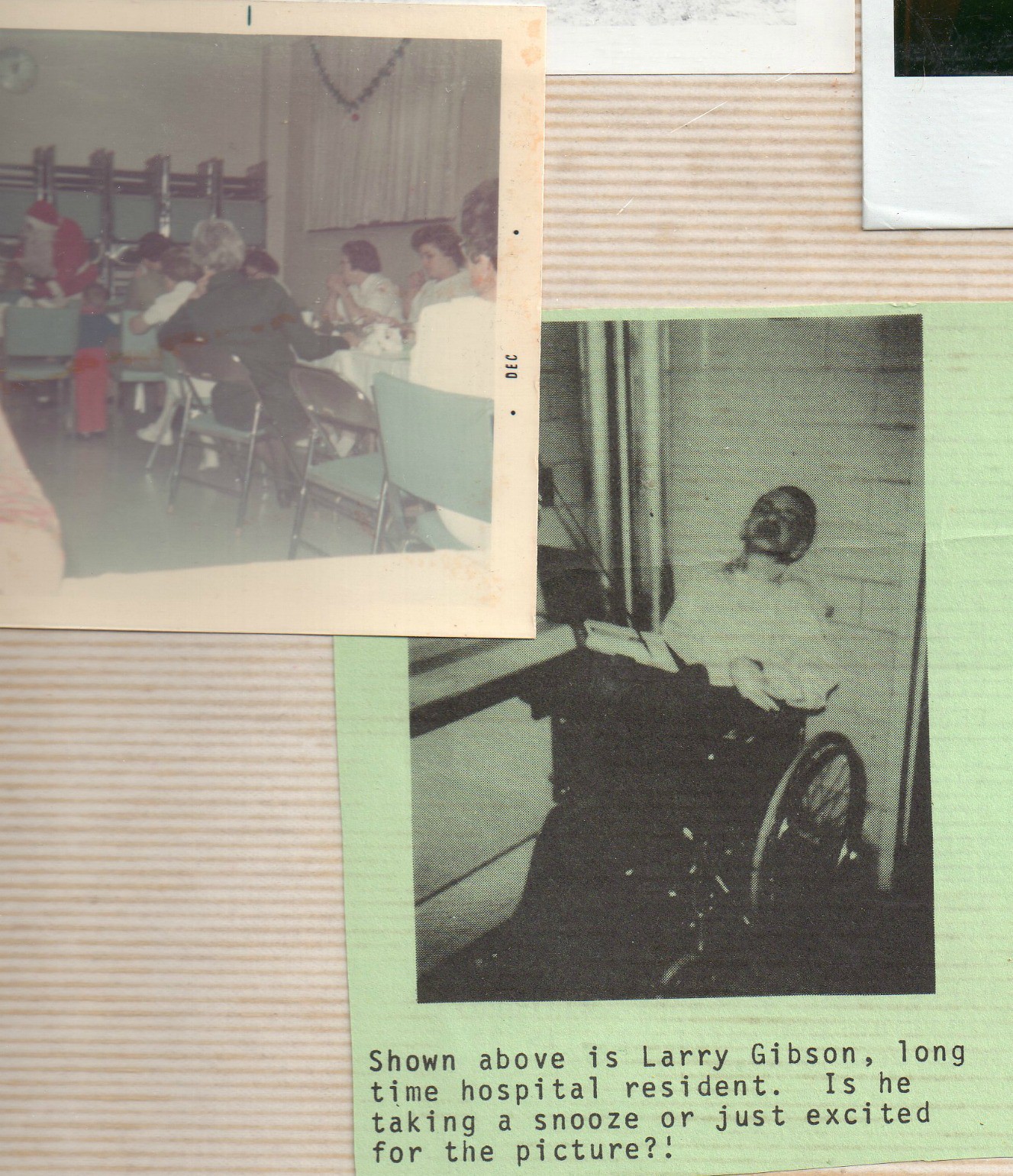The image showcases what appears to be a part of a photo album, evident from the sticky background typical for such albums. At the top left, there is an old Polaroid photograph bordered in white and marked with "DEC." This picture is somewhat faded and blurry but depicts a festive scene with a Santa Claus figure dressed in a red and white suit standing in the foreground, accompanied by a child nearby. Around them, several women are seated at long banquet tables draped in white tablecloths and flanked by silver metal chairs with green cushions. 

Below this, there is another picture reminiscent of a newspaper clipping. This black-and-white photograph, set against a green background, shows a man named Larry Gibson, a longtime hospital resident, lounging in a wheelchair. He appears to be either asleep or deeply relaxed with his eyes closed, leaning back against a stone wall. The caption below reads: "Shown above is Larry Gibson, longtime hospital resident. Is he taking a snooze or just excited for the picture?"